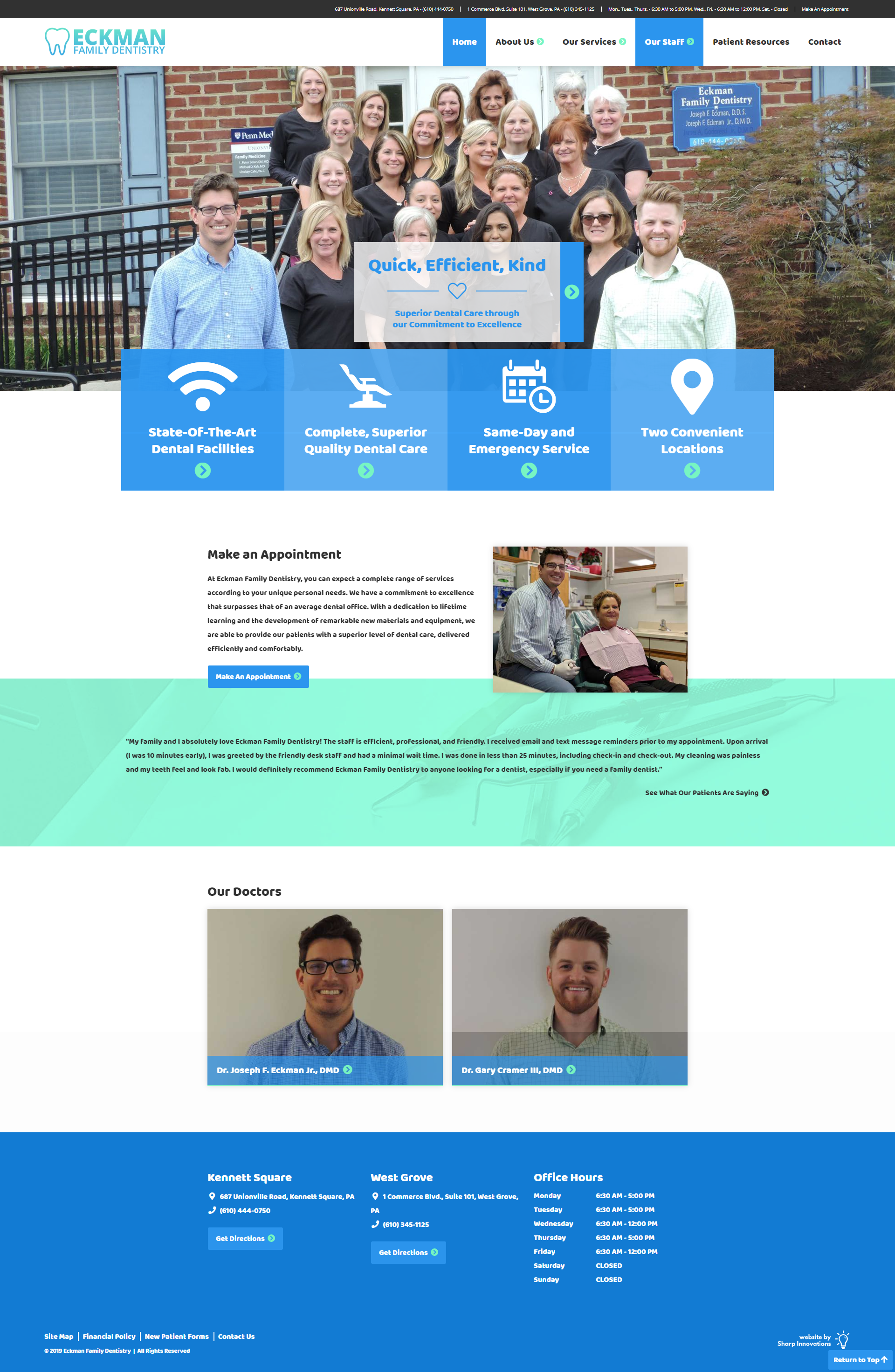The image depicts a full-page view of a website for Ekman Family Dentistry. Due to the extensive vertical scroll, the content appears quite small. Starting from the top, a slim horizontal black bar spans the width of the screen, containing white text that is unfortunately illegible given the zoom level. Below this, a thicker horizontal white bar occupies approximately 5% of the screen's height. On the left side of this white bar, the Ekman Family Dentistry logo is featured in teal, showcasing an outlined tooth, alongside the text "Ekman Family Dentistry."

On the right side of the white bar, there is a navigational menu with the items: Home, About Us, Our Services, Our Staff, Patient Resources, and Contact, all written in black except for Home and Our Staff, which are distinguished by a light blue background and white text. 

Beneath the white bar, a prominent banner occupies nearly a quarter of the screen's height. This banner contains a group photograph presumably depicting the dental clinic's staff. The group consists primarily of women, with the exception of two men positioned at the front corners of the group. They are standing in front of a brick building with a railing, all smiling warmly. The individuals appear to be in their 30s or 40s, providing a welcoming and professional introduction to the team at Ekman Family Dentistry.